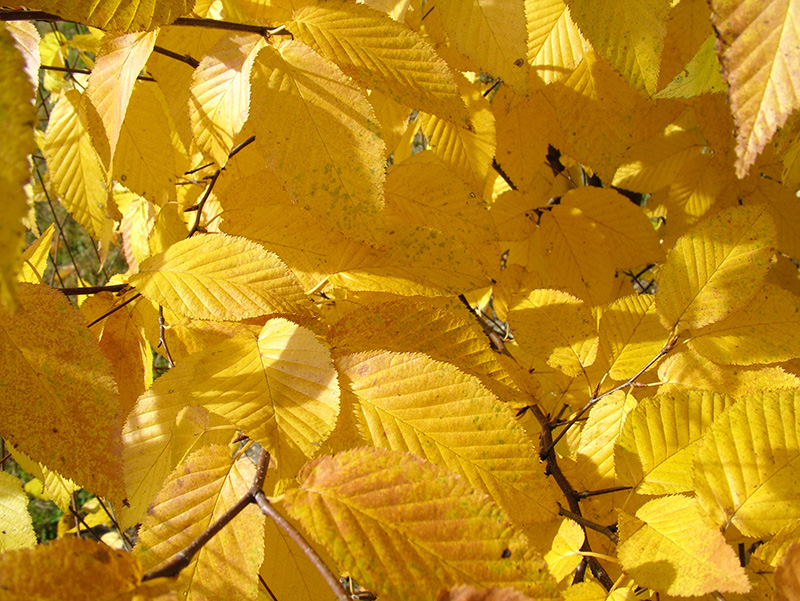The image captures a densely packed assortment of yellow and orange leaves, creating a rich tapestry that fills the entire frame. These slightly oval-shaped leaves display a vibrant mix of mustard yellow with hints of orange and gold, indicative of the fall season. Shadows from the overlapping leaves are cast across the scene, enhancing the depth and texture of the arrangement. In the left 20% of the image, a blurry patch of green suggests the presence of grass peeking through. The composition appears somewhat staged, as the leaves are arranged in various directions, covering the ground in a dense mat. Despite some areas appearing almost natural, there are no visible stems or clear background elements, making the photograph an immersive study of autumn foliage. The interplay of light and shadow, along with the diverse palette of fall colors, suggests that the image could be the work of a professional photographer, though it might also have been captured with a standard camera.